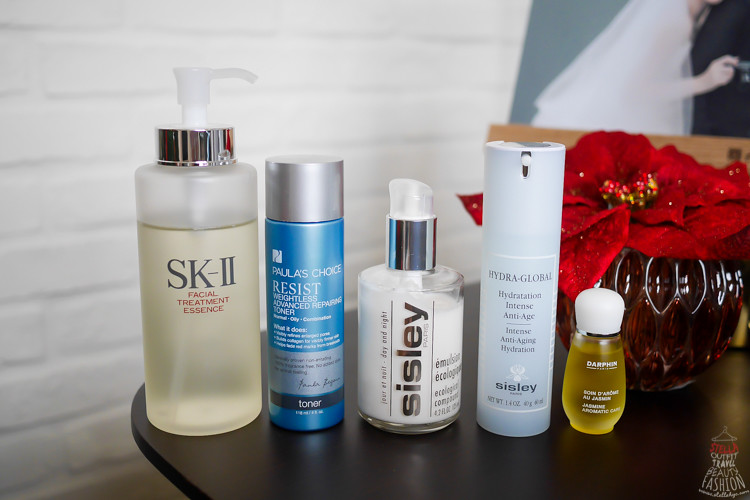The image depicts a detailed skincare routine setup. From left to right, the array includes:

1. **SK-II Facial Treatment Essence**: A signature product known for its skin-renewing properties.
2. **Paula's Choice Resist Weightless Advanced Repairing Toner**: This toner is formulated to repair and refresh the skin.
3. **Sisley Emulsion Ecologique**: Designed for both day and night use to hydrate and protect the skin.
4. **Sisley Hydra-Global Intense Anti-Aging Hydration**: This intensive hydration product aims to combat signs of aging.
5. **Aromatics Elixir**: A small yellow bottle containing a scent known for its rich and complex aroma.

The collection showcases a blend of premium skincare products aimed at maintaining and enhancing skin health.